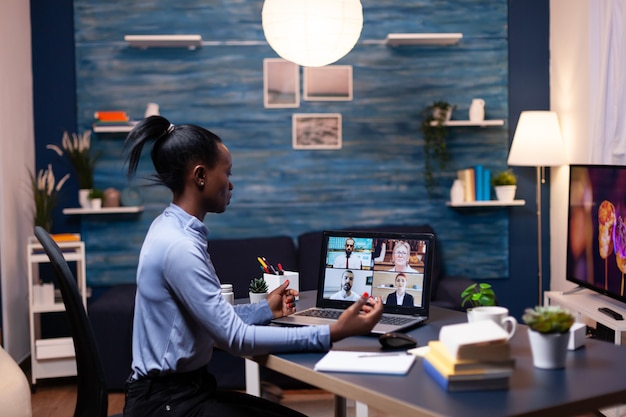In the image, a young black woman is meticulously working from what appears to be a home office. She is sitting at a dark-colored desk, engaged in a Zoom call displayed on her computer screen, which is divided into four sections with three men and one woman—comprising a black man, two white men, and a white woman—participating in the discussion. Her workspace is neatly organized with a variety of items, including two small plants, a stack of books, a white coffee mug, a notepad, and a pen. Additionally, a small succulent plant and a white pen holder cube are positioned on her left side.

The room is predominantly medium blue, adorned with shelves and three pictures on the wall behind her. A round overhead orb light illuminates the space. The office further features a lamp with a white shade on the floor, next to a flat screen TV located on the right side of the wall. A small bookcase can be seen on the left-hand side of the image. She is seated in a black chair, and there is a blackish couch towards the back. She is casually dressed in a blue, college-style shirt paired with black pants. The overall ambiance suggests a well-organized and inviting remote work environment.